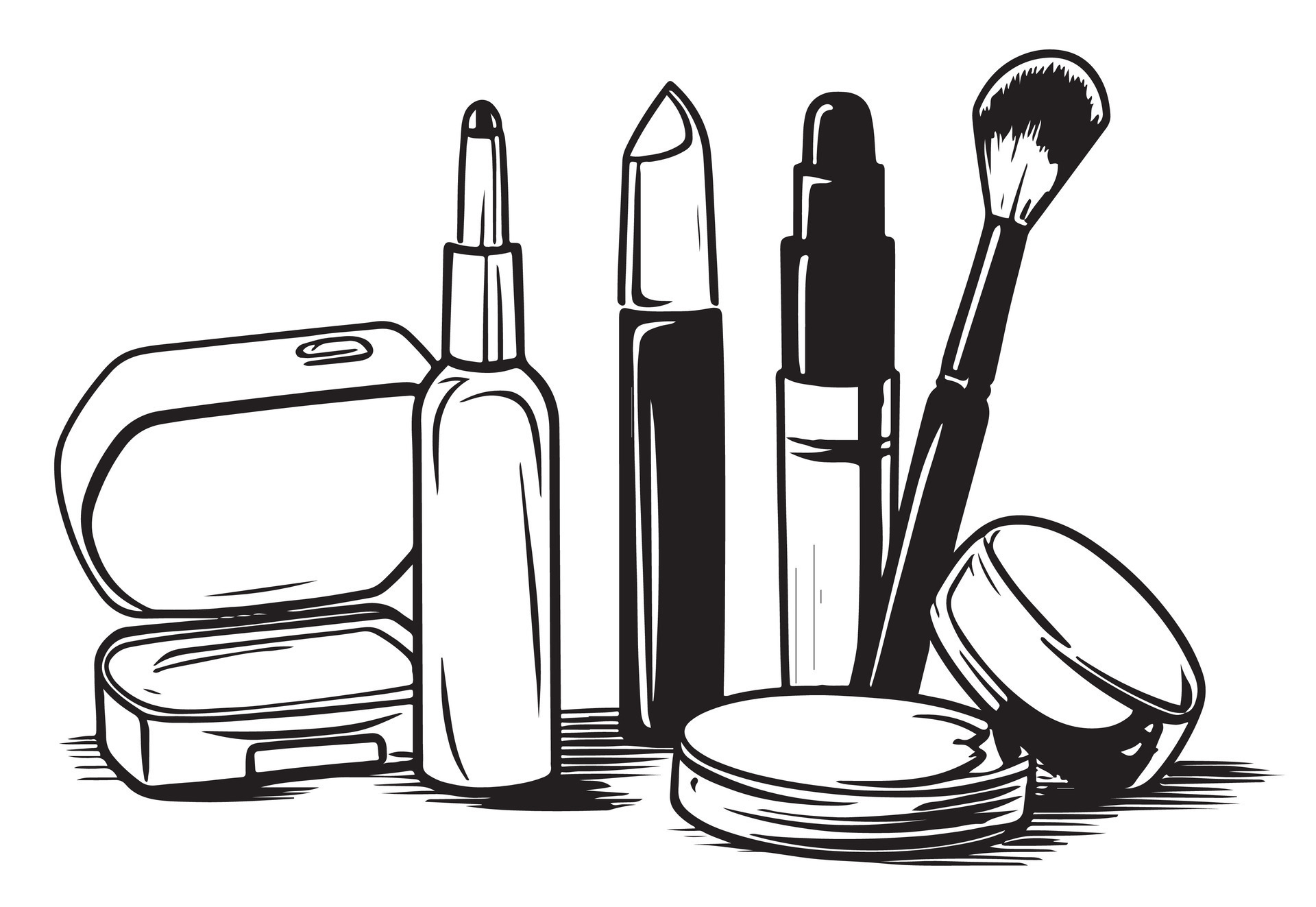This detailed black and white line drawing showcases an array of cosmetic items, effectively capturing shadows with dense black lines against a whitish background. On the left, there is an open compact likely featuring a mirror and powder. Adjacent to it, an unlabelled small bottle resembling an eyedropper stands next to an upright lipstick, which has a black tube and a contrasting white top. Further right, a white vial with a black top is followed by a makeup brush angled slightly, its bristles defined in black. Completing the scene is a small tin, possibly holding powder, which is open and meticulously illustrated. The objects are outlined in black with several having areas shaded almost entirely black, except where light reflections are indicated by precise white lines. This minimalist depiction focuses on the essential details and silhouettes, making each cosmetic item easily recognizable.